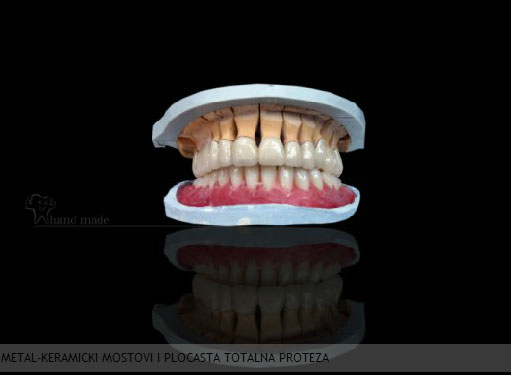The image depicts a detailed, computer-rendered model of a human mouth, set against a stark black background, featuring both upper and lower teeth held within a light blue plastic mold. The upper teeth are held together by a bronze object protruding from the blue plastic, and the lower teeth are set into pink gums. The teeth themselves are a pearly off-white color with beige roots. An inverted reflection of the teeth appears beneath the model, creating the illusion that the teeth are resting on a reflective surface. Text in another language, saying "metal, keramichi, mostavi, plocasta, totalna, proteza," is written on a horizontal light gray bar at the bottom of the image, with a watermark labeled "handmade" positioned at the middle left.